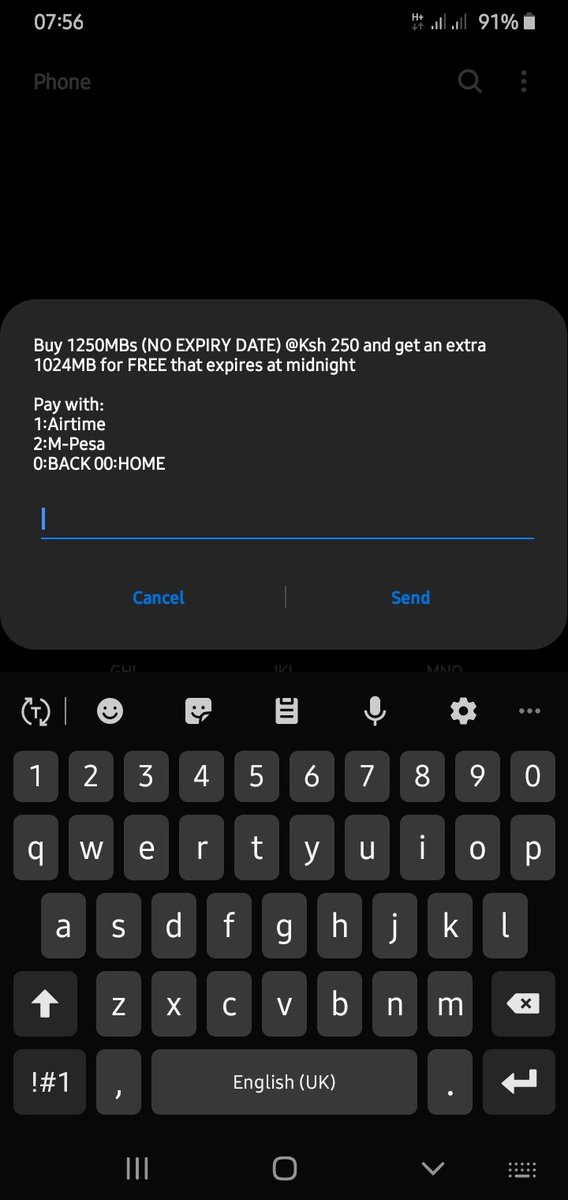In this image, the time displayed at the top of the screen is 7:56. Below the time, there is a mobile phone interface showcasing a pop-up offer. The pop-up message reads: "Buy 1250 MB with no expiry date at KSH 250 and get an extra 1024 MB for free that expires at midnight." Users are presented with several payment options: "Pay with airtime (1)," "M-PESA (2)," "Back (0)," and "Home (0)." There are also two buttons at the bottom of the pop-up, "Cancel" and "Send," both highlighted in blue. The on-screen keyboard is black with white letters, and it includes several emojis: two smiley faces, a rectangular-shaped notepad emoji, a microphone emoji, and a settings emoji.